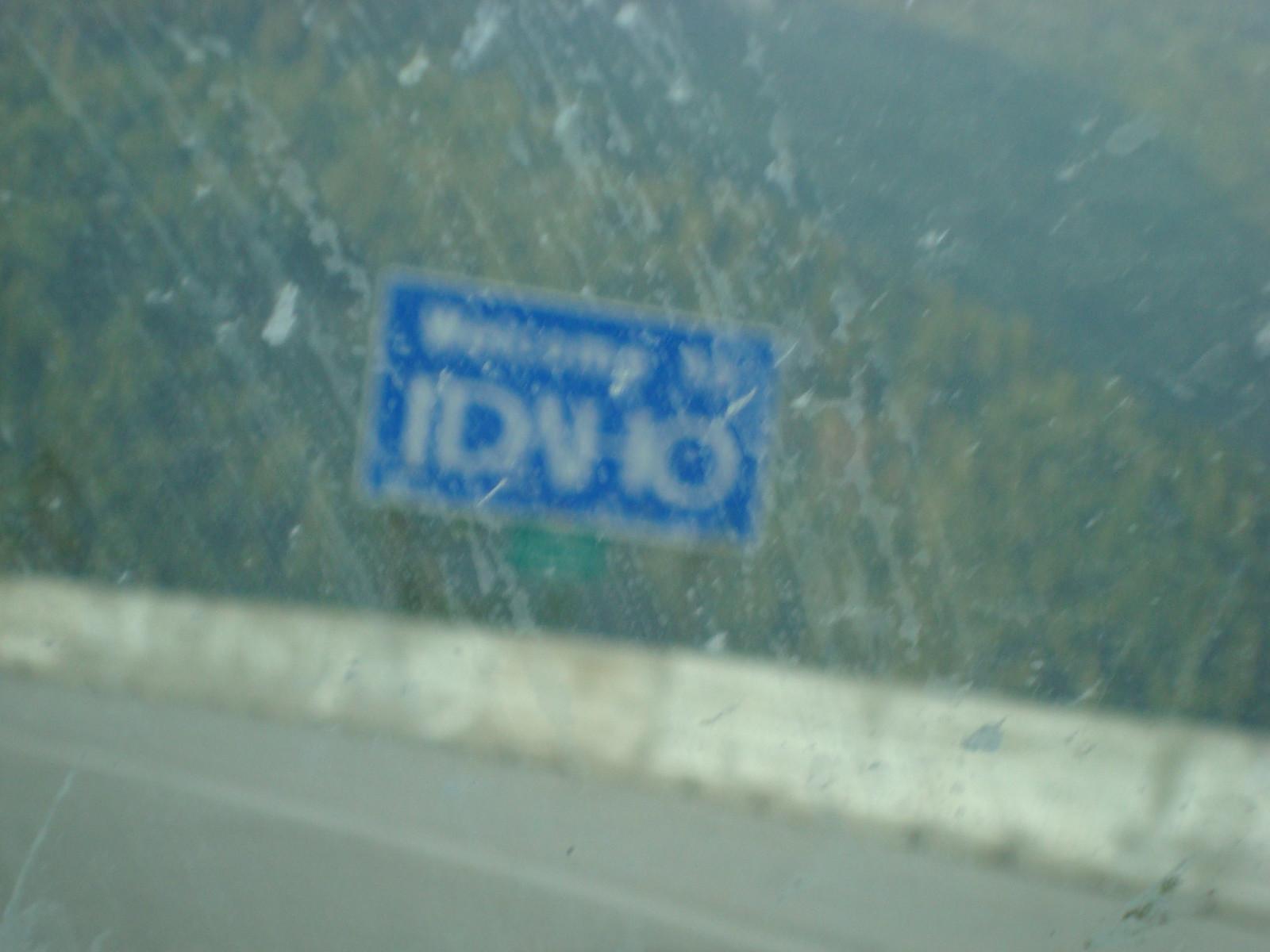The photo, taken from the inside of a very dirty car through the front windshield, captures a gray asphalt road. The windshield is marred with numerous white splatters and streaks from an ineffective use of windshield washing fluid and wipers, resulting in a blurred and streaky view. Ahead on the road, a large blue rectangular sign with a white border, mounted on two stilts, reads "Welcome to Idaho." Despite the blur, the text is discernible. In the background, a substantial hill or mountain covered in dense forest rises, suggesting that the road traverses a higher elevation, possibly through foothills or a mountainous region. Adjacent to the road is a concrete side barrier adding to the sense of altitude and terrain.